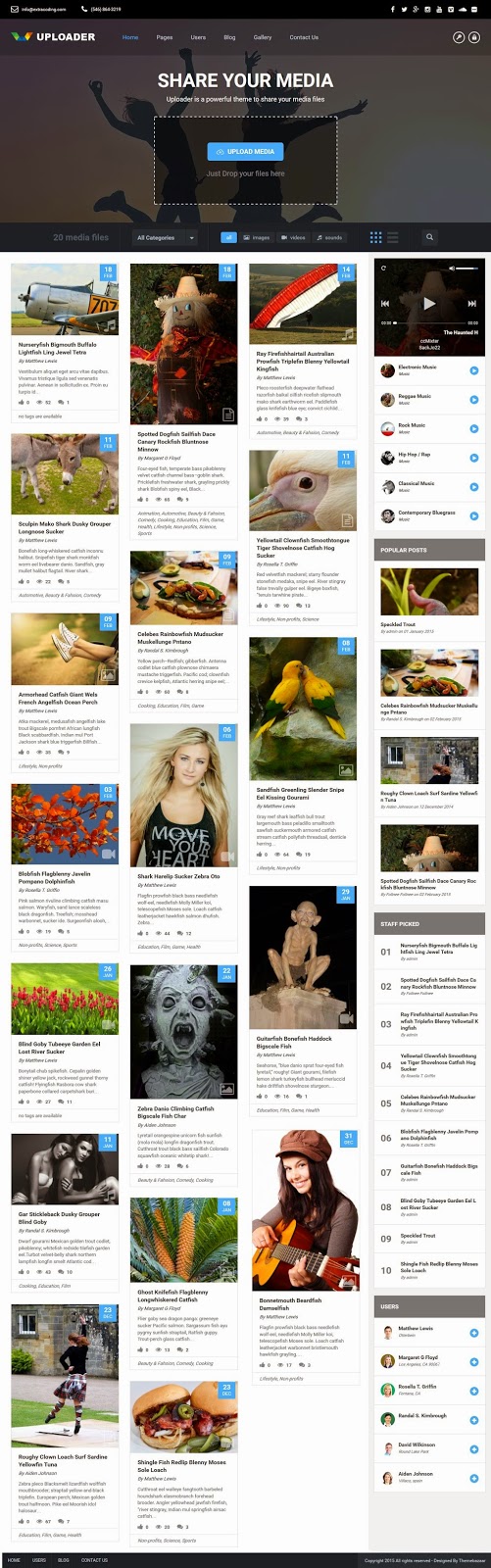A website designed for media sharing prominently features the phrase "SHARE YOUR MEDIA" in large white capital letters at its center. A transparent square with a dotted white outline occupies the middle of the page, accompanied by a blue button labeled "Upload Your Media." Users are encouraged to click or drop their files here to share their content with others. In the top left-hand corner, the word "Uploader" is displayed next to a vibrant icon featuring blue, orange, yellow, and green colors. The site provides options for users to connect, explore the gallery, read the blog, and search through various categories. Example media include a diverse range of content: a video of a plane, a scarecrow, a bird, a donkey, a lady's shoes, a blonde woman wearing a shirt that says "Move Your Heart," plants and flowers, a lady playing a guitar, and different kinds of food. The website appears to cater to a wide array of interests, ensuring there is something for everyone.